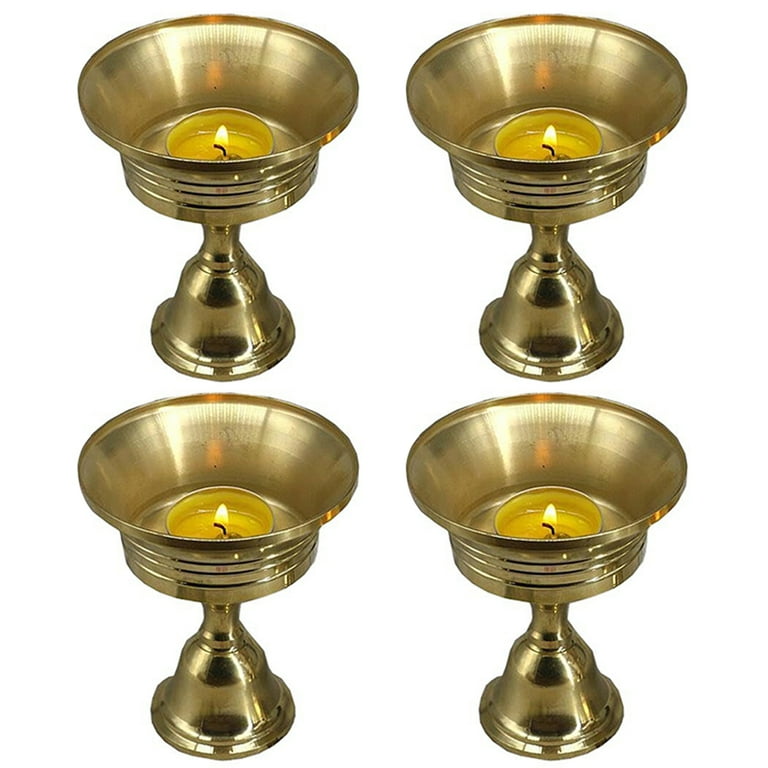This photograph, seemingly taken for a shopping website, presents four identical candle holders arranged in a 2x2 grid against a spotless white background. Each holder, resembling a goblet or chalice, features an elegant silver or brass finish with a wide, bell-shaped base that narrows upward before flaring out to a broader, lip-edged cup. The design includes three etched lines around the cup area, adding a touch of intricate detailing. In each holder, a tea light candle is placed, all of which are lit, showcasing short wicks and mostly melted wax with small yellow flames flickering. The reflective surface of the holders captures subtle lighting highlights, emphasizing their polished and sophisticated appearance.